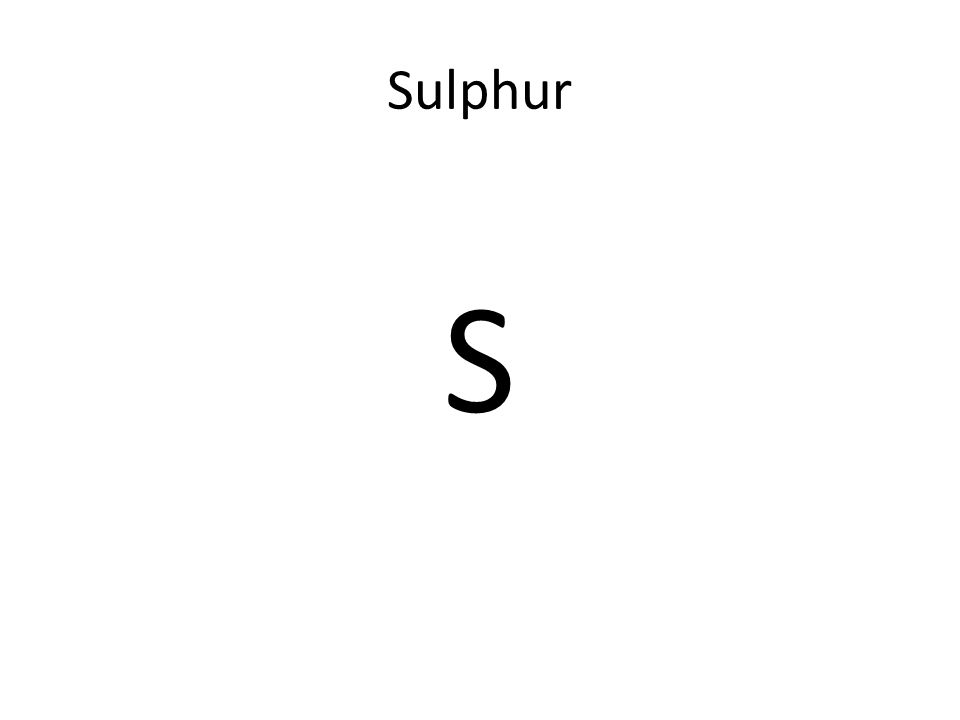The image features a stark white background with just two elements of black text. At the top, the word "Sulfur" is displayed in capital letters ("SULFUR"), centered and in black text. Below it, positioned towards the middle of the image, there is a bolded capital letter "S," also in black. Both "Sulfur" and the "S" are precisely centered with respect to each other. No other elements such as images, references, or colors are present, creating a minimalist and clean composition. The layout suggests it could be an educational or scientific graphic, possibly related to the periodic table.